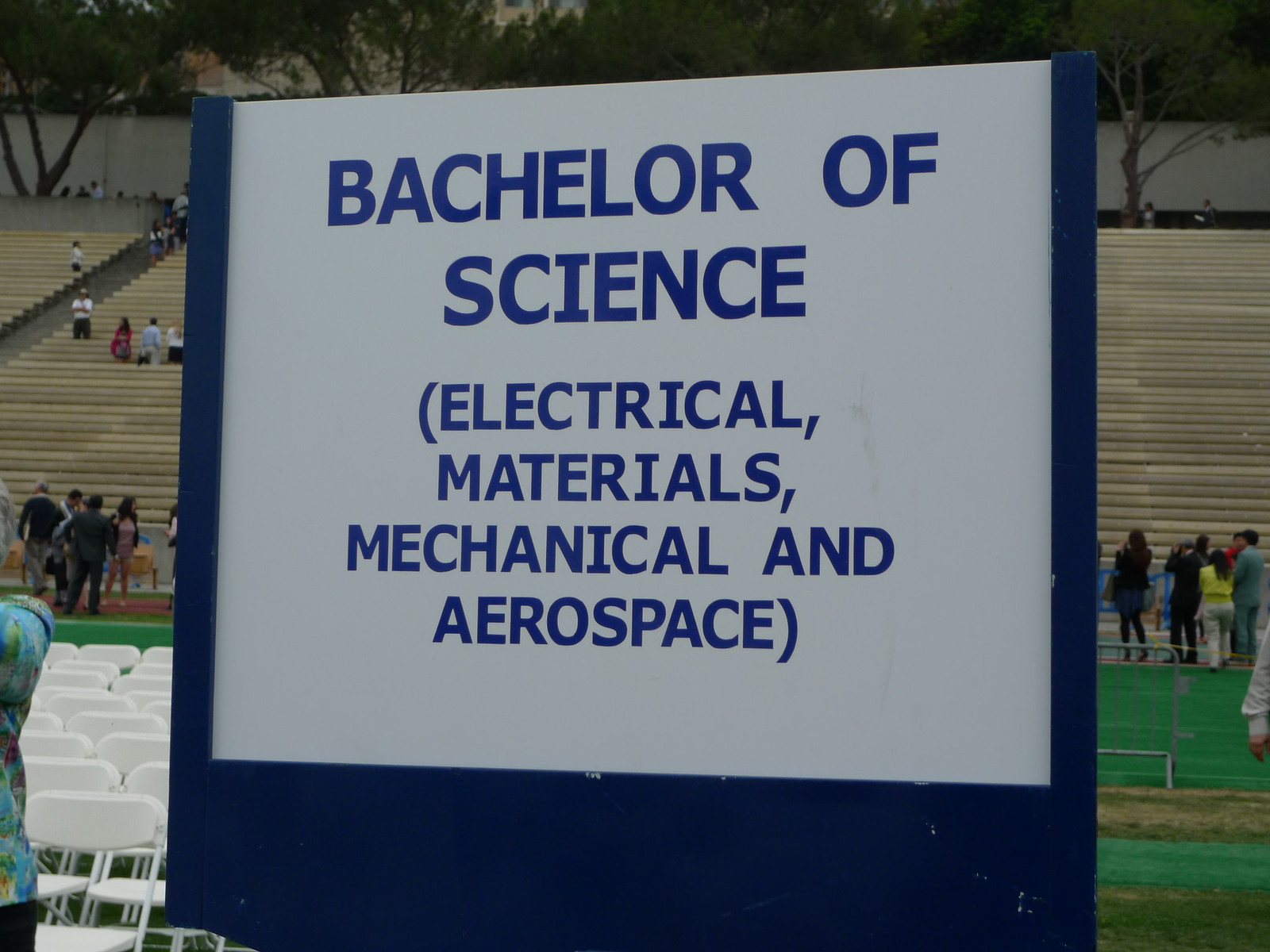The image captures an outdoor scene, likely at a school or stadium field, perhaps set up for a graduation event. Dominating the foreground is a sign made of blue-painted wood with a white background. The sign prominently displays in blue text: "Bachelor of Science, Electrical Materials, Mechanical and Aerospace." To the left of the sign, a row of white folding chairs is neatly arranged, while in the background, more white lawn chairs are visible, stacked next to each other. The backdrop features a grassy area and large bleachers built along a hill, with people scattered across them, some of whom are taking pictures behind metal railings. Above the bleachers and the ongoing activity, lush green trees frame the top of the scene, adding to the outdoor ambiance.